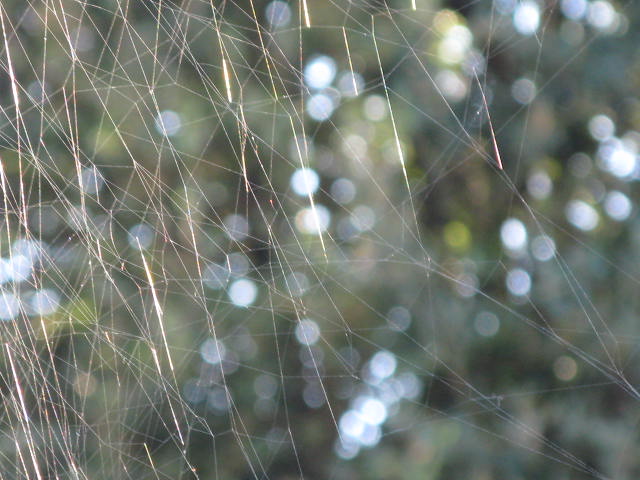This close-up photograph captures the intricate beauty of a spiderweb suspended in an outdoor setting. The web, which spans the entire frame, diverges from the traditional circular pattern. Instead, it forms a complex array of geometric shapes through interwoven strands that densely cluster in the lower left-hand corner before fanning out with larger spaces toward the upper and lower right-hand corners. The background remains indistinct, shrouded in a mosaic of rich green hues, suggesting an outdoor environment but leaving specific details to the imagination.

Sunlight enhances the web's gossamer threads, giving them an almost ethereal, see-through quality. Additionally, the photographer’s choice of lens introduces small, vibrant blue and white circular flares across the image. These flares, alongside the reflection of what appear to be water droplets on the web, add a professional touch and a dreamy atmosphere to the composition. Although the proximity of the shot obscures the exact nature of the background flora, the interplay of light and natural elements ensures the spiderweb remains the focal point, compelling in its delicate complexity.